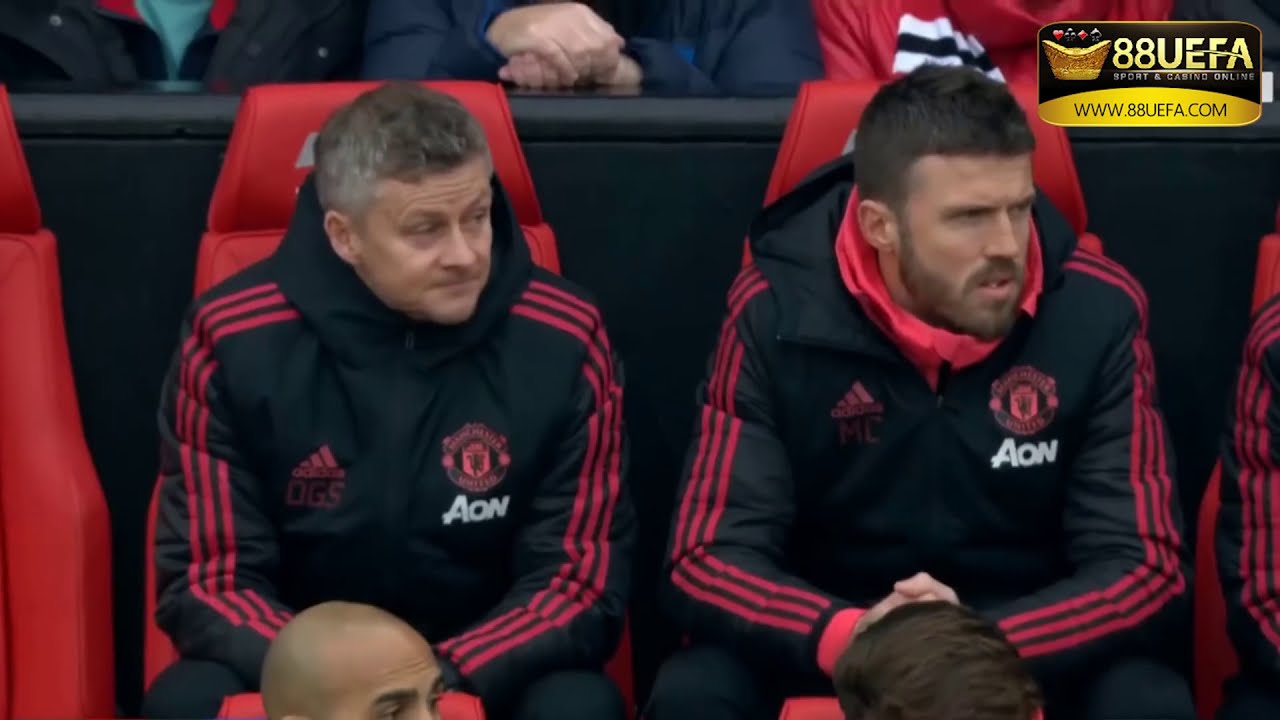The photograph captures an audience at a sports event, focusing primarily on two men seated next to each other in red leather chairs. Both men are wearing identical black Adidas jackets with red accents, featuring the AON logo on the right chest. Their postures are nearly identical, leaning slightly forward with their forearms resting on their thighs, and they are both looking towards the right. The setting appears to be a spectator section, with several people partially visible both behind and in front of them. In the upper right corner of the image, a black and golden icon is visible, displaying the text "88UEFA Sports and Casino Online" alongside the URL "www.88UEFA.com."